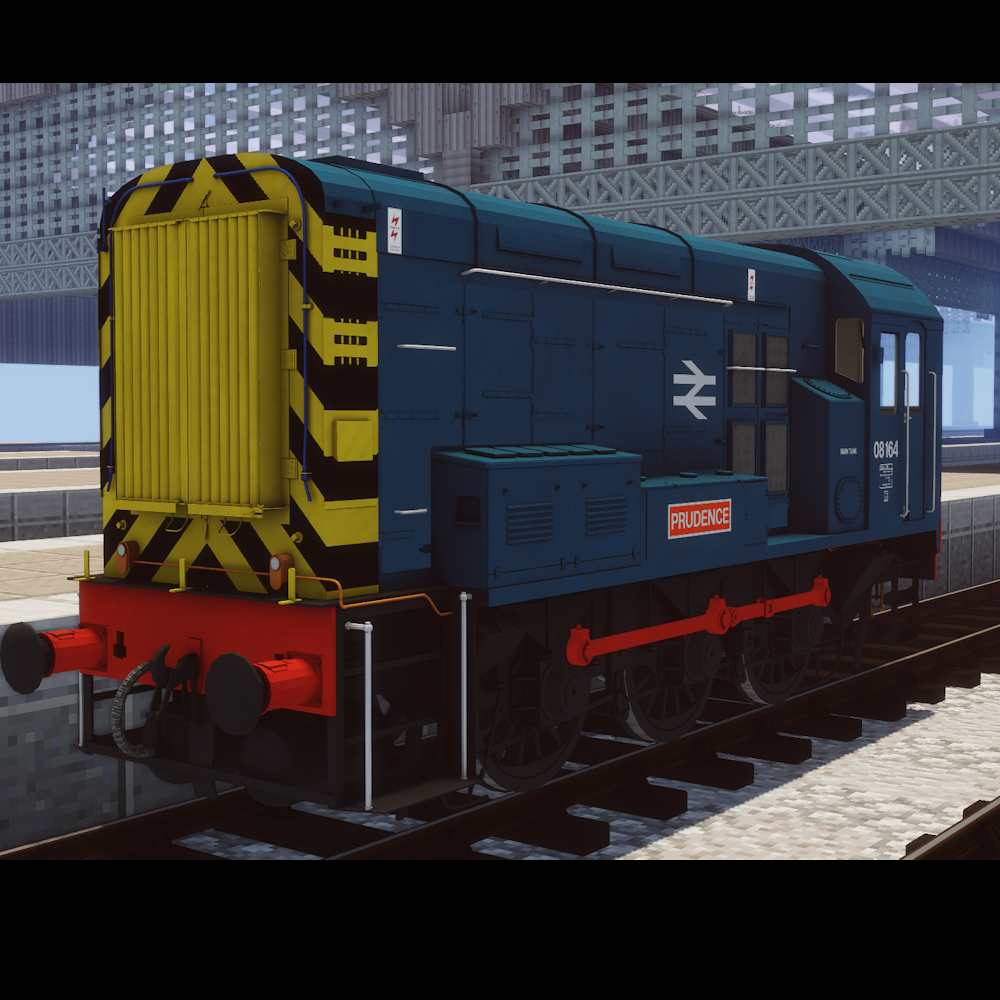The image depicts a highly detailed, computer-generated train engine within a station setting. The square-shaped image, approximately 5 to 6 inches on each side, features a black border framing the scene. The train engine, primarily blue with metal panels, vents, and step ladders, sits on dark brown and gray metal train tracks over a pixelated, gray concrete base. Notably, the front of the train, facing left, sports bright yellow and black caution chevron patterns, particularly around the vented grill area. A prominent red sticker with the text "Prudence" in white is affixed to the blue side of the engine. The engine also includes a red bumper plate with two black bumpers, and its wheels and gears are black with a connecting red bar. The station environment includes an elevated platform on the left and a white floor on the right, as well as a building with numerous windows that appear gray to greenish in color. The overall scene emphasizes the realistic textures and complex details typical of high-quality video game graphics.